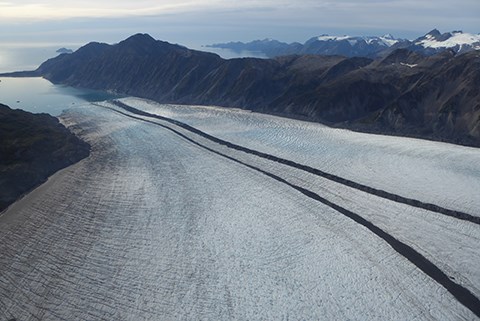The photograph captures a breathtaking mountain landscape in a horizontal layout, with the scene perfectly encapsulating the raw beauty of nature. Dominating the upper portion of the image is a hazy blue sky, partially obscured by a blanket of white clouds. In the distance, beneath the cloud cover on the right, looms a series of stone mountains with peaks crowned in pristine white snow. Closer to the viewer, the dark, almost black mountains create a stark contrast against the brighter background.

At the center of the landscape, a glacier stretches out, its snowy surface marked by visible tire tracks that meander towards the distant valley. The glacier appears to be the central feature of the scene, surrounded by rugged rock formations particularly noticeable on the left, where a black triangular landmass protrudes into the frame.

In the lower left corner, a serene lake mirrors the sky above, with its waters possibly partially frozen, giving an unusual coloration. Intriguingly, towards the right of the center, the terrain splits into another section of water, suggesting a complex network of mountain ranges and bodies of water interspersed throughout the scene.

Overall, this composition vividly highlights the juxtaposition of the tranquil lake, the rugged, rolling mountains, and the imperfect, human touch of tracks etched into the glacier.